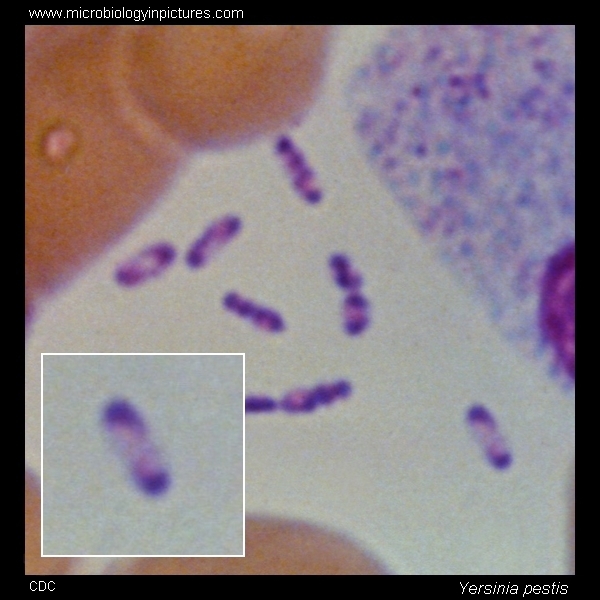This image appears to be a detailed microbiological photograph taken through an ultramicroscope, showcasing the bacterium Yersinia pestis. The photograph is framed in black, with "www.microbiologyinpictures.com" written in white text at the top left and "CDC" along with "Yersinia pestis" at the bottom right. The central focus of the image is a collection of purple, pill-shaped bacteria, resembling microscopic creatures. These bacteria appear to surround an orange cell-like structure. There is an inset close-up in the bottom left that highlights one of these bacterial cells in more detail, displaying a gradient from dark to light purple along its length.